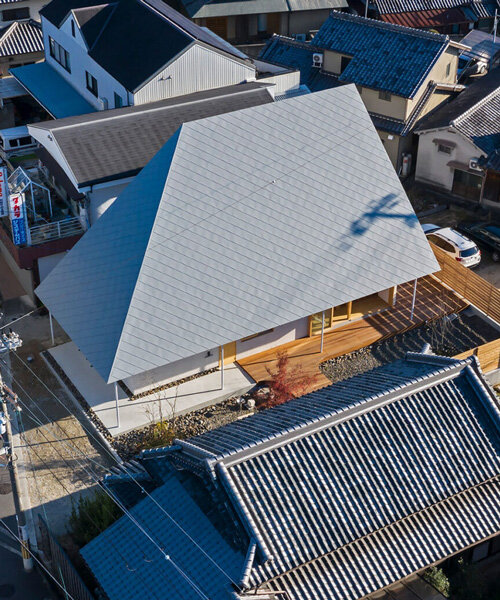This aerial photograph captures a clustered neighborhood, showcasing a distinctively unusual, high-pitched gray roof that serves as the image's focal point. This gray, triangular roof, with subtle ridgelines, overhangs its house to the extent that the house itself is barely visible, only hinting at a yellow facade beneath. Surrounding this modern and sharply angular roof are more typical houses with average roofs, including a notable blue shingle roof and another with regular gray shingles. The scene is detailed with visible power lines crisscrossing the area and a street below where a white car is parked. To the left, there’s a small sign with Asian writing, suggesting the location might be somewhere in Asia. The neighborhood is built on varying elevations, with the intricate wooden decks and teak-like sidewalks enhancing the residential setting. Additionally, the upper left area appears to host more commercial structures, contrasting with the primarily residential surroundings.